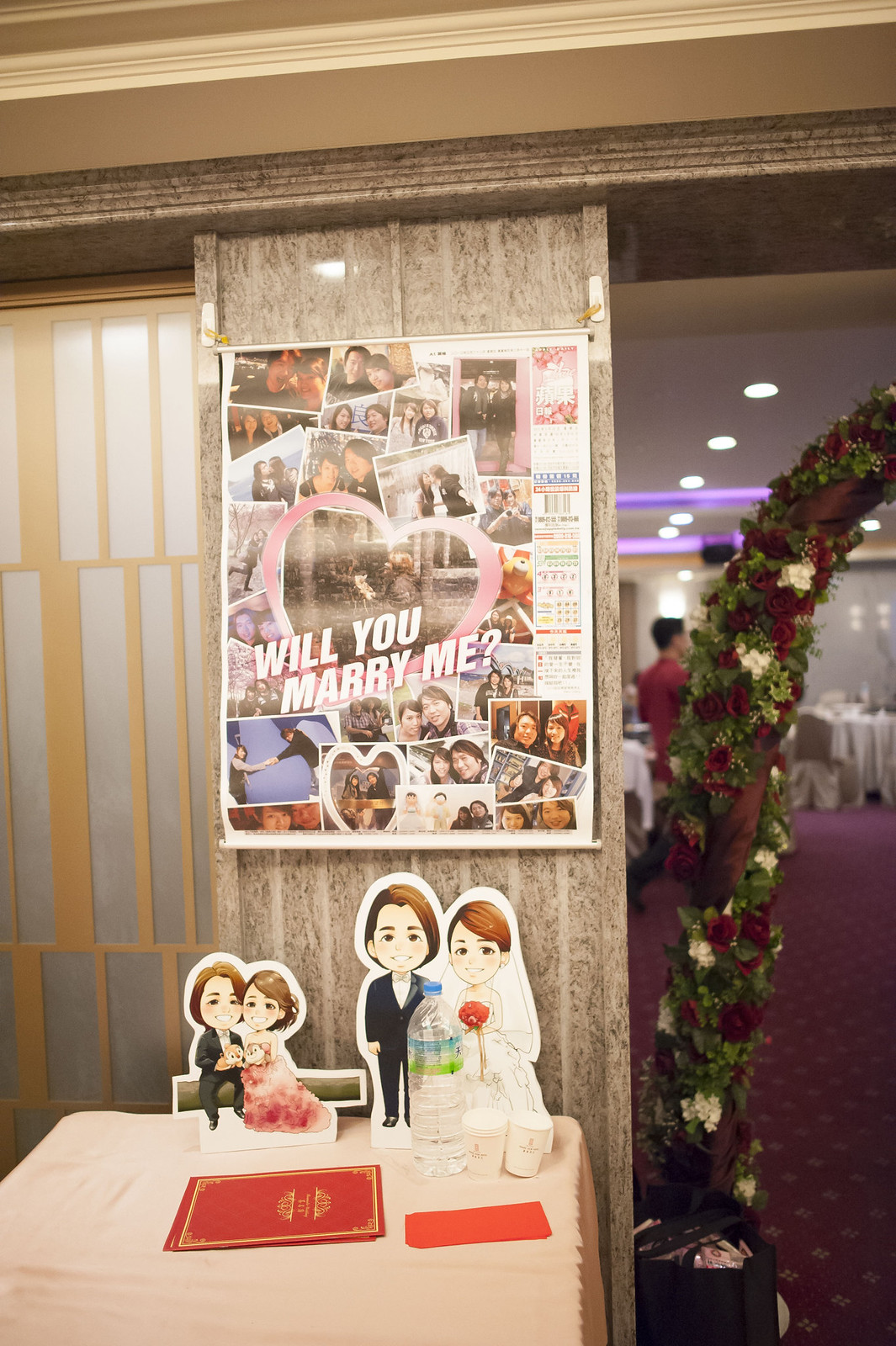The image depicts an elaborate marriage proposal or wedding reception setting. Central to the scene is a table adorned with a pink tablecloth, upon which rests a red napkin, a red menu, a water bottle, and some cups. Prominently displayed above the table is a large poster bearing the words "Will you marry me?" along with a pink heart. The poster features a collage of photos showing an Asian couple in various poses, including kissing, sitting together, and holding hands. Beneath the poster are cardboard cutouts of the couple, depicted twice: once with the man in a black suit and the woman in a pink dress, and again with the man in a black suit and the woman in a wedding dress holding a bouquet. Completing the romantic atmosphere, an archway decorated with flowers stands nearby, enhancing the intimate and celebratory vibe of the scene.